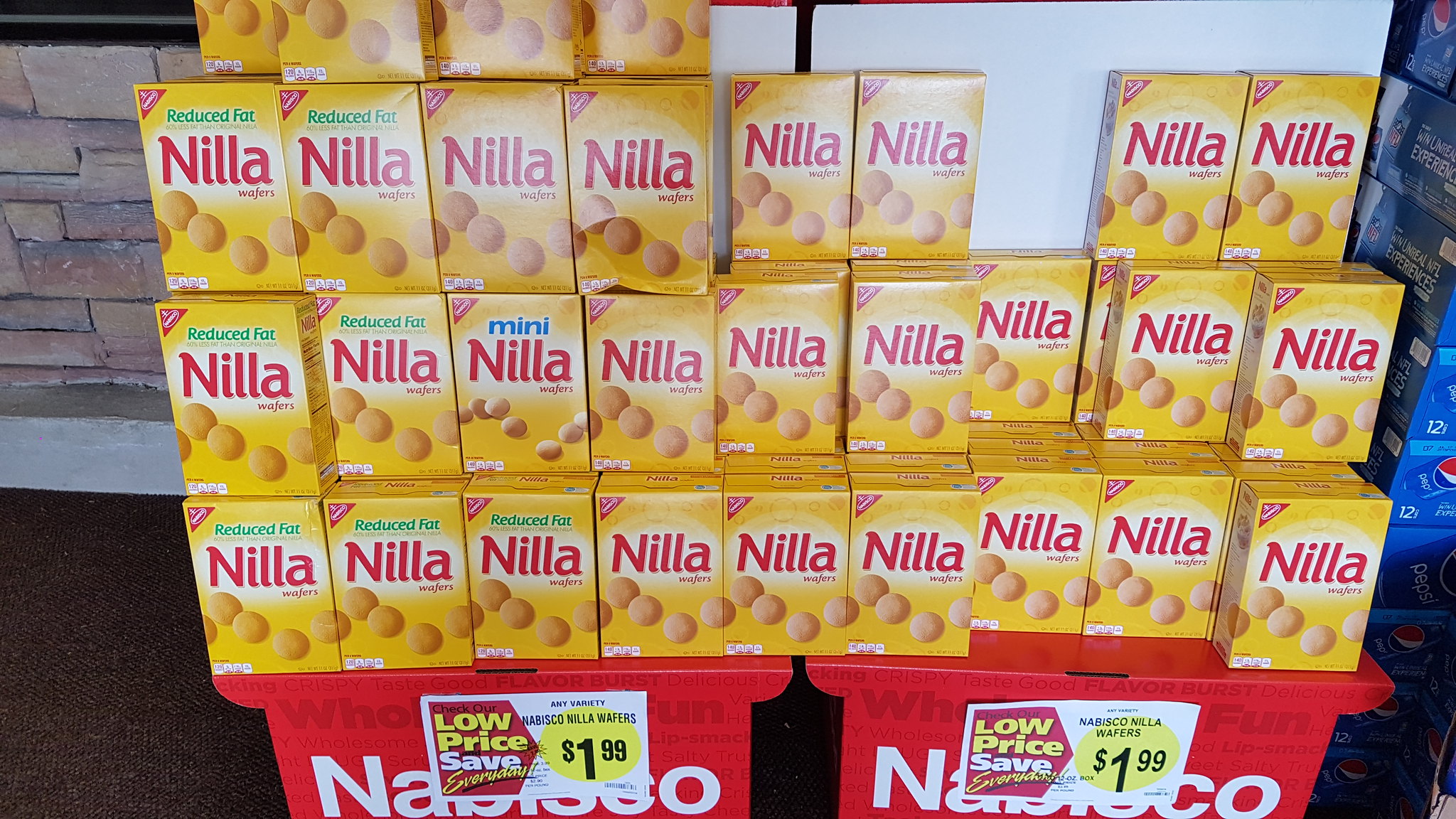This color photograph captures a detailed display likely set up in a grocery or convenience store. Centered prominently are two large red stands adorned with white Nabisco lettering, partially obscured by signs touting a low price of $1.99. These stands support four orderly rows of Nabisco’s iconic yellow Nilla wafer boxes. 

The boxes include three variations: the standard Nilla wafers, reduced-fat Nilla wafers in three vertical stacks on the far right, and a single box of Mini Nillas tucked between rows. Each standard box showcases the red Nilla logo, red Nabisco emblem in a white oval, and images of four vanilla wafers.

Positioned beside the displays is a stack of 12-packs of canned Pepsi, colored in signature blue, red, and white, evoking a lively store ambiance. To the left, a brick wall with hues of brown, red, and gray adds a rustic texture, while concrete flooring and a hint of brown indoor-outdoor carpet ground the scene. Behind the setup, a partially visible window hints at the indoor setting. This image meticulously captures the strategic arrangement and vibrant branding aimed at attracting customers.